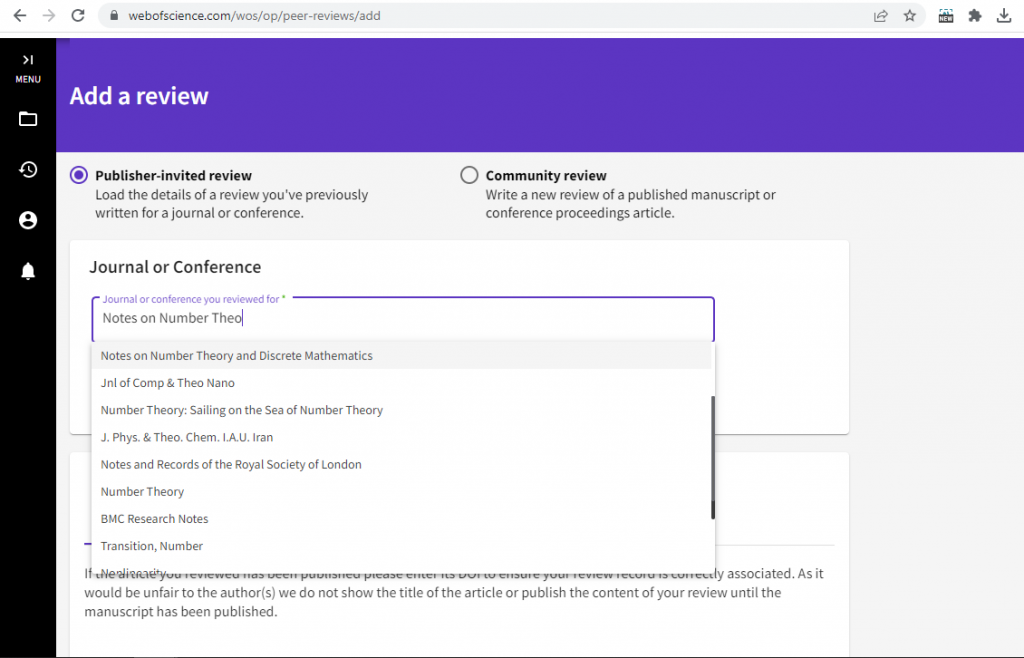The photograph captures the interface of a webpage from the website webofscience.com, specifically at the URL: webofscience.com/WOS/OP/peer-reviews/add. At the very top, a gray navigation bar includes a back and forward arrow alongside a refresh button, followed by a secure (padlocked) search bar. Additional options to favorite, forward, and download the webpage are also available within this bar.

Below the navigation bar, a prominent purple banner announces the function of the page: "Add a Review". To the left of the page, a vertical sidebar labeled "Menu" displays icons for a folder, refresh, profile, and notification bell.

Central to the webpage, under the purple "Add a Review" banner, is the section titled "Publisher Invited Review". This section contains a selected radio button inside a purple circle. The description reads: "Load the details of your review you've previously written for a journal or a conference."

Adjacent to this, there is an unselected radio button under the heading "Community Review". The description here states: "Write a new review of a published manuscript or conference proceedings articles."